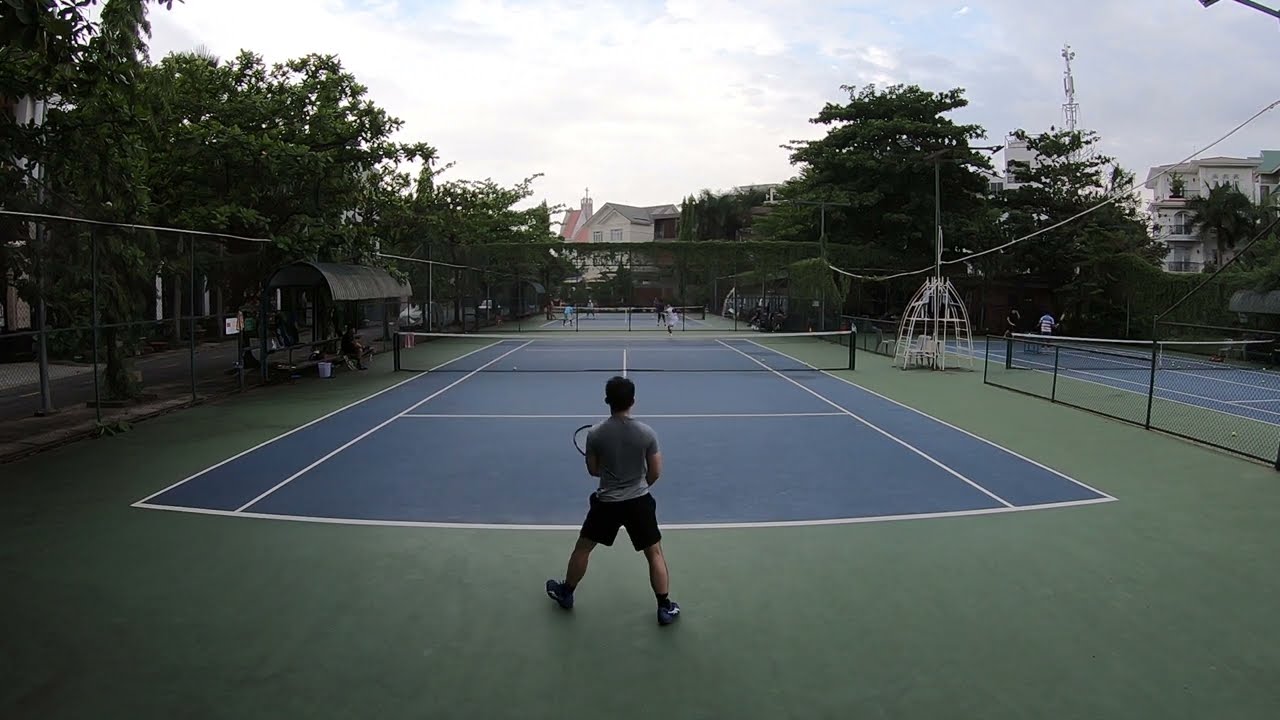The image depicts an outdoor tennis court framed by a dark green walkway and enclosed by a black chain-link fence. The court itself is blue, with clear white lines marking the various play zones and edges. In the center, two green pillars support a black net with a white top. The scene is set under a mostly cloudy sky with glimpses of light blue. In the distance, there are multi-story, rectangular white buildings.

The focus is on a young man, likely in his 30s or 40s, standing on the green part of the court, with his feet apart and slightly bent in a ready stance, gripping his racket. He wears a gray shirt and black shorts. Across the court, someone dressed predominantly in white stands on the odd side, poised to serve. The setting suggests this is a park with multiple tennis courts; neighboring courts are visible, separated by shorter chain-link fences.

To the left, there is a covered area with benches and several individuals seated, shaded by thick trees lining the street outside the facility. The right side features a referee's white structure and some white, three-story apartment buildings surrounded by more trees. The overall atmosphere is gray and overcast, as if a storm is impending, lending a sense of urgency to the players keen to finish their match.